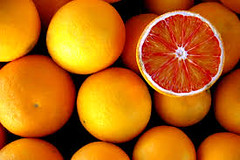This is a low-res square photograph depicting a cluster of round citrus fruits against a black background. At first glance, these fruits appear to be oranges due to their smooth, uniform skin and varying shades of orange and yellow. However, upon closer inspection, one fruit in the top right corner is cut open, revealing the red flesh and triangular segments characteristic of a grapefruit rather than an orange. There are approximately 15 fruits visible, slightly varying in color, with some showing a brighter yellow hue which could either be a trick of the light or an indication of different types of citrus. The dark void behind and between the fruits accentuates their vibrant colors, creating a stark contrast that highlights their spherical shapes and smooth peels. The image seems to be a stock photo, perhaps depicting a display of these fruits in a box, though the box itself is not visible.